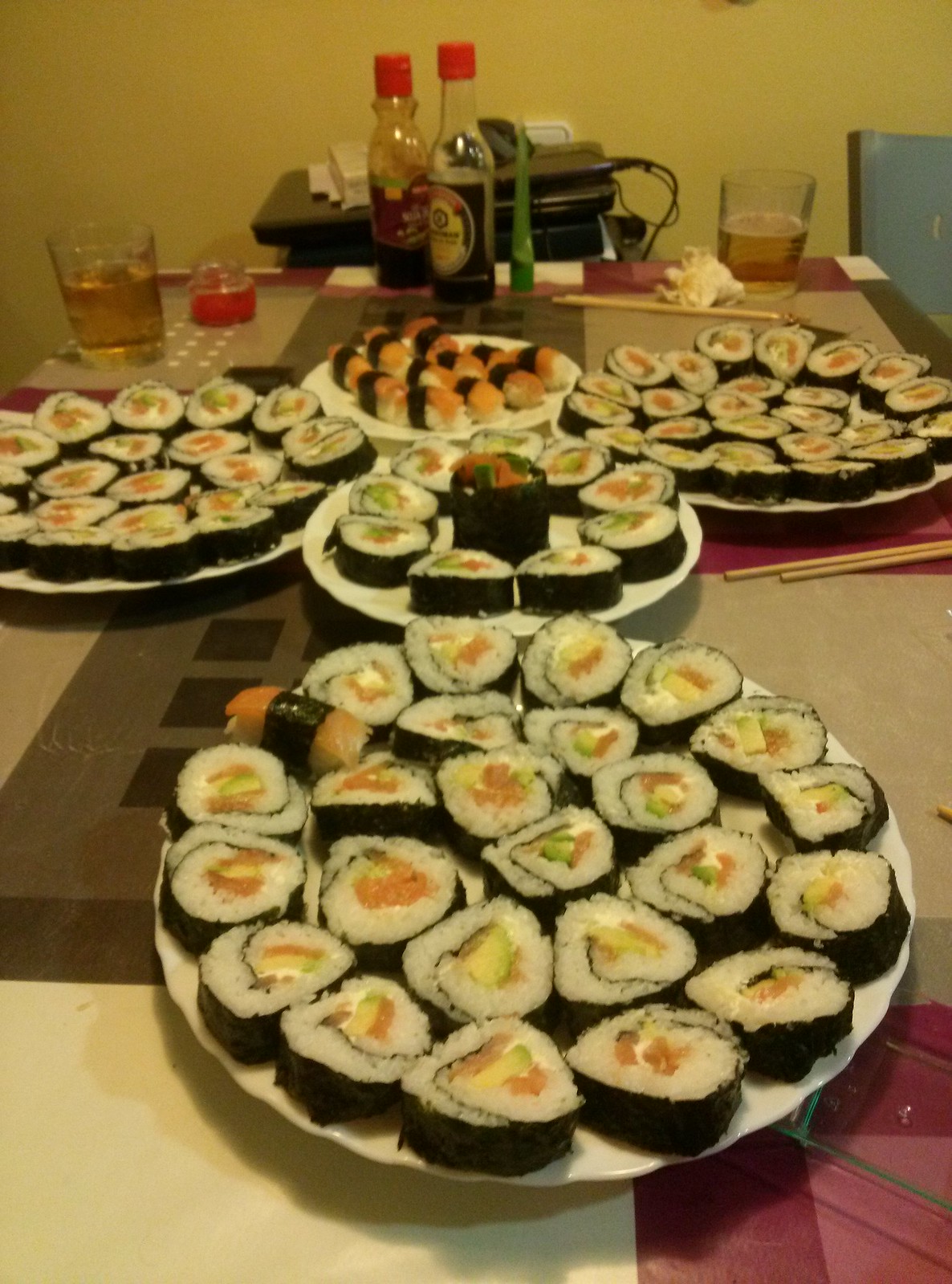This image portrays a neatly arranged dining setting featuring five white plates of sliced, round sushi rolls. Four of these plates display sushi rolls with a black outer layer, a white inner layer, likely filled with fish, green vegetables, and possibly avocado, suggesting they might be California rolls. The fifth plate presents sushi with an orange-hued filling, also wrapped in black seaweed. All the plates rest atop a table covered with a vibrant tablecloth, adorned with large gray, pink, and purple squares in a distinct pattern. 

On the right side of the table lie two sets of chopsticks, while in the background, two bottles of condiments with red tops are visible—the shorter one on the left and the taller one on the right, likely soy sauce and another similar condiment. Additionally, there are two glasses filled with a pale liquid, one positioned on the left and the other on the right, resembling either beer or apple juice. A small glass on the left contains a red liquid or sauce. This visually appetizing setting suggests a cozy meal either at a restaurant or a home dining table, ready for an enjoyable sushi experience.